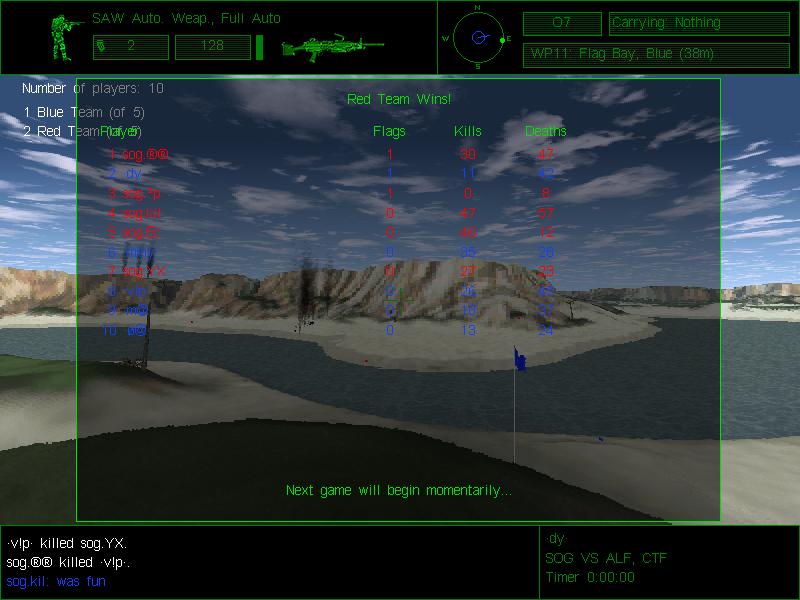This screenshot from a video game captures a post-game leaderboard, set against a scenic background featuring light brown and tan mountains, a light tan and beige sandy foreground, and a grayish-blue river. The sky is a vivid blue with white clouds scattered throughout. On the left side, a splotch of green is visible on another sandy beach across the river. Dominating the center is a large rectangle with an opaque black background and a green border, displaying game results. At the bottom of this rectangle, text announces, "Next game will begin momentarily." The scoreboard within shows the results for multiple players, detailing flags captured, kills, and deaths, with names like SOG, DY, SOQ, LIL, and GOG featured. Notably, the red team is declared the winner. Additionally, there's a silhouette of a character holding a gun on the left side, labeled with "SAW AUTO WEAPON FULL AUTO" and a small icon depicting a saw. A compass indicating northwest, east, and south is also present above the black rectangle.